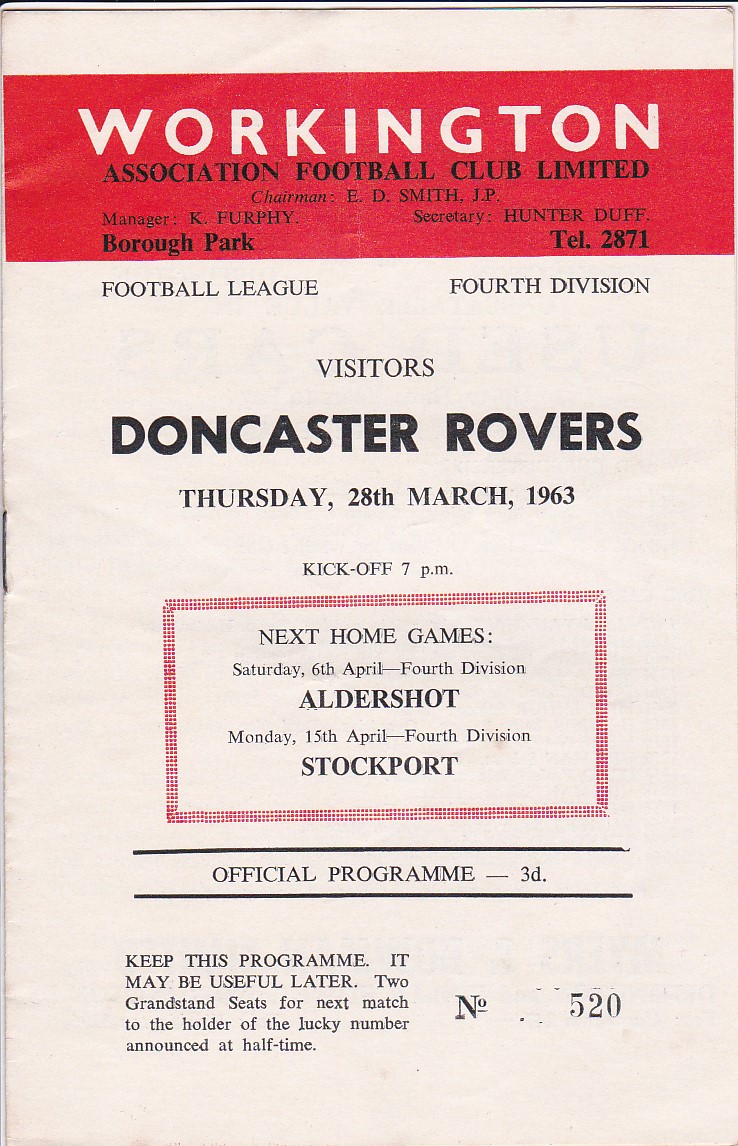This vertical rectangular photograph displays the cover of an official program for an upcoming soccer match. At the very top, it features a horizontal red rectangular band with the white text "Workington" prominently displayed. Directly beneath in smaller black letters, it reads "Association Football Club Limited." Additional details such as "Chairman E.D. Smith, J.P.," "Manager K. Farfi," and "Secretary Hunter Duff" are listed alongside the club's address, "Borough Park, TEL 2871."

The main white section of the program cover contains black text, beginning with "Football League 4th Division" to the left and "Visitors" followed by "Doncaster Rovers" to the right. The date "Thursday 28th March 1963" and the kickoff time "7 PM" are prominently placed in the center.

Below this, a red-bordered box outlines information regarding upcoming matches, with details such as "Next Home Games: Saturday 6th April - 4th Division Elder Short" and "Monday 15th April - 4th Division Stockport." The program is labeled "Official Programme - 3D" just below a black separation line, with a notice at the bottom urging readers to "Keep this Programme; it may be useful later." It mentions a special offer of "two grandstand seats for the next match to the holder of the lucky number announced at halftime," with the current program featuring the number "520."